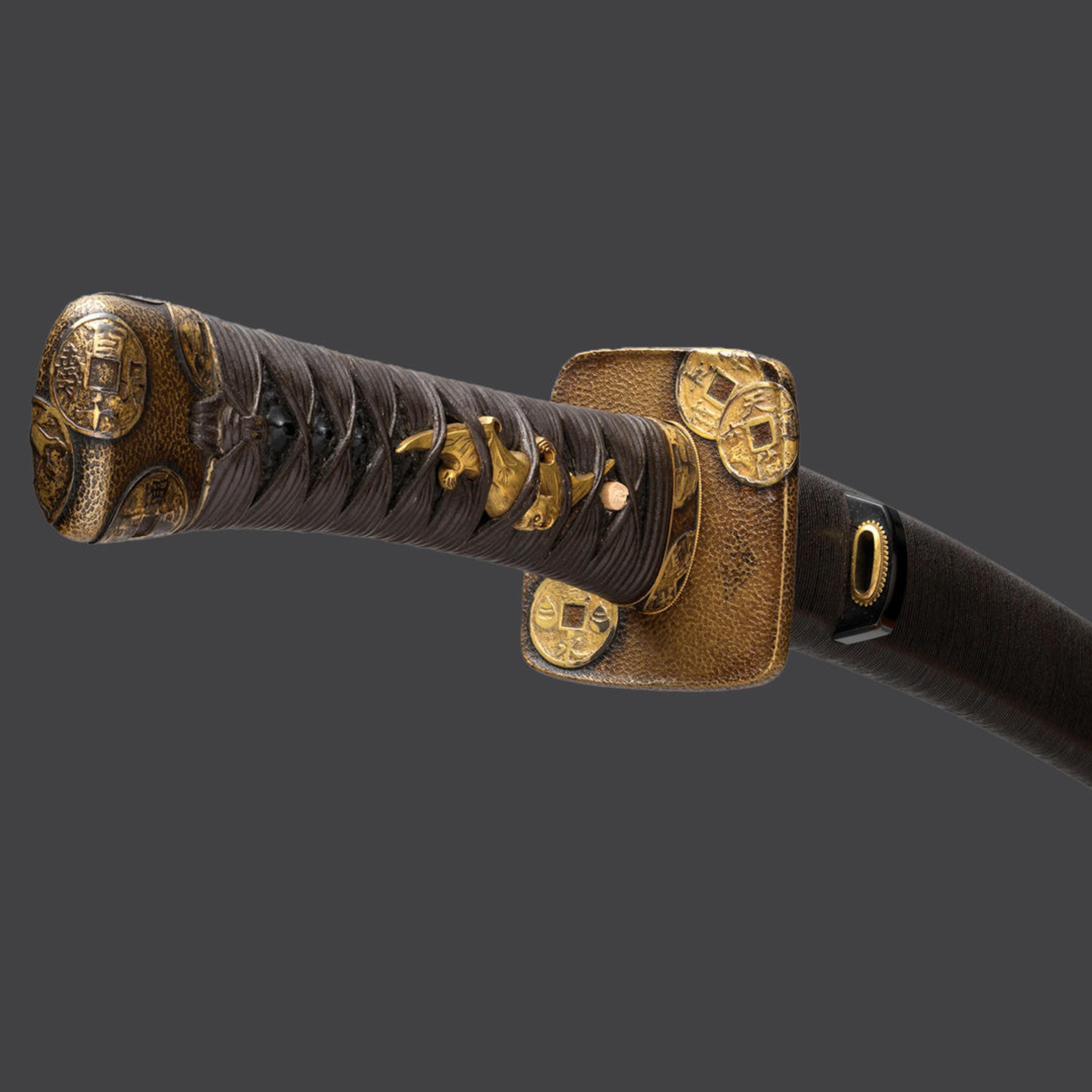The photograph depicts the central handle of an ornate sword, likely a katana, with elaborate craftsmanship that appears to be quite ancient, potentially hundreds of years old. The handle, which is primarily gold or copper in color, is intricately wrapped with gray metal wire and adorned with emblems and symbols, including motifs resembling old coinage. The handle transitions into a sheathed blade, with the sheath extending from left to right across the image, exhibiting a dark black leather look with gray trimming. The entire sword is positioned against a plain gray background, highlighting its detailed design and craftsmanship. Despite the sword's awe-inspiring and imposing appearance, there is no text visible within the image to provide further context.